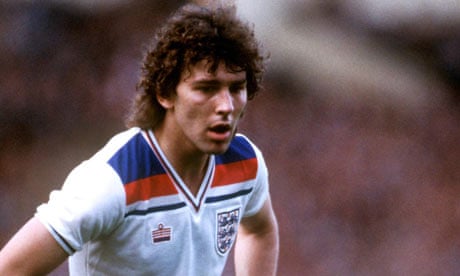The image captures a male soccer player of Hispanic appearance with tan skin and brown, curly hair that falls to the nape of his neck and reaches the top of his shoulders in the back, tapering off around his ears on the sides. The athlete is the focal point of the photograph, which is in color and landscape format, with a completely blurred background that ensures all attention is directed towards him. He dons a white, short-sleeved V-neck jersey adorned with red, blue, and black stripes across the shoulders. Prominently displayed on his chest are two emblems: a team emblem on the right side and a smaller flag emblem on the left. The player’s expression is one of surprise or perhaps exhaustion, with his mouth slightly open as if catching his breath. The detailed composition and the athlete's focused yet incredulous demeanor capture a moment of intensity, possibly from a thrilling match.